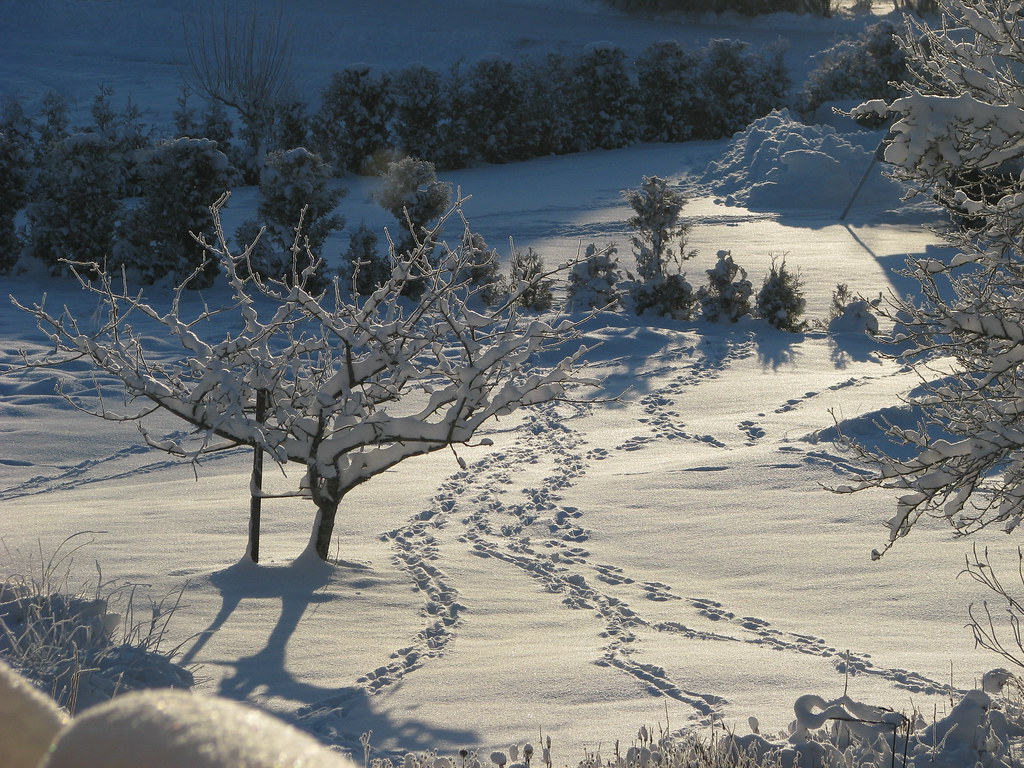The image is a landscape-oriented, color photograph capturing a serene, snow-covered hillside at night. From the bottom of the image, a series of three to four distinct paths of animal footprints meander up towards the center, eventually converging and then diverging again. The entire landscape is bathed in the gentle glow of moonlight coming from the top right, casting a serene, almost magical atmosphere. On the left side, a barren, leafless tree stands laden with a heavy coat of snow, mirrored by a similar snow-covered tree on the right. At the far end, a row of stout, green pine trees encircles the hillside, each branch weighed down by a blanket of snow. Small shrubs pepper the landscape, adding texture and depth to the pristine snowy field. The overall scene is one of tranquil beauty, with the moonlight highlighting the intricate details of the snowy terrain and the delicate patterns of the animal tracks.